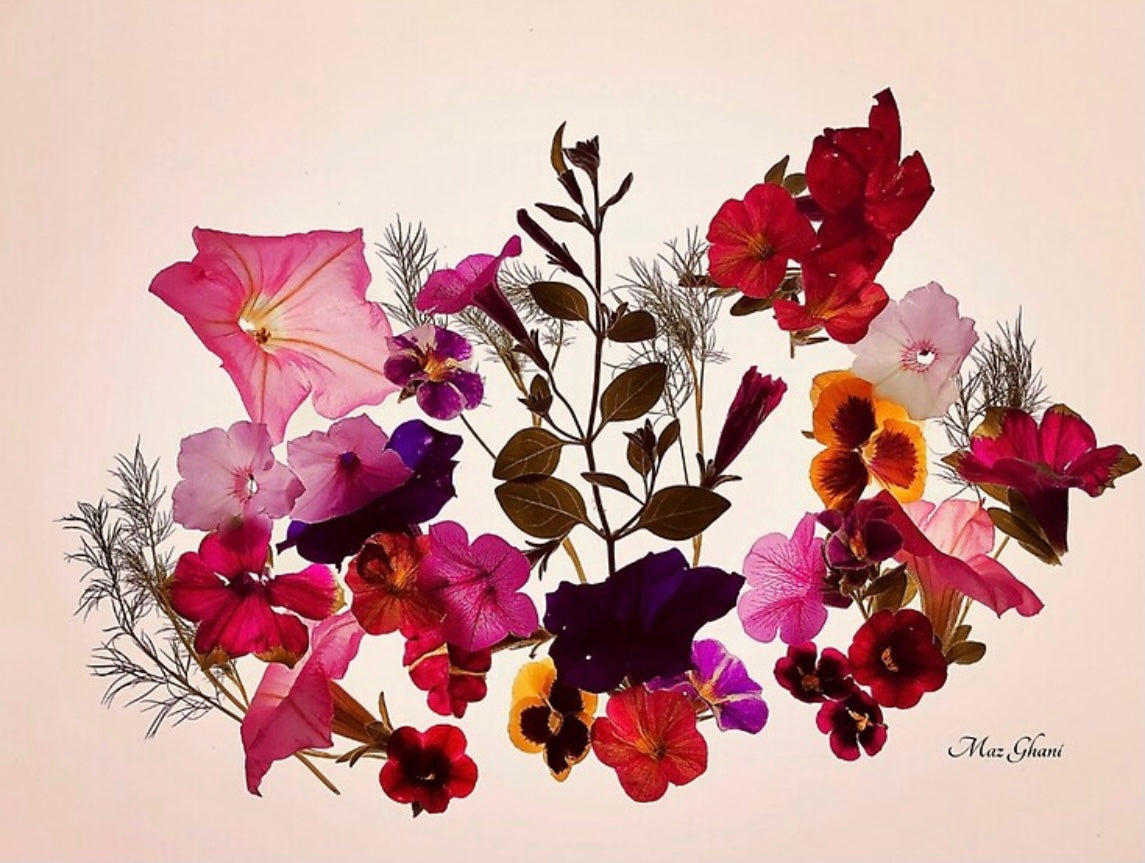This piece of art, signed by the artist Maz Ghani at the bottom in elegant italic text, portrays a bouquet of flowers with a blend of photographic realism and artistic interpretation, possibly rendered in pen and ink or watercolor. The background is a very light peach with hints of pink and gold, providing a luminous backdrop that enhances the vivid colors of the flowers. The bouquet features a diverse array of flowers in shades ranging from red, dark pink, and purple to yellow, with some flowers displaying intricate color variations like yellow centers with red or pink edges. The flowers appear translucent under bright lighting, highlighting their fragile textures and different shadings. Interspersed among the colorful blooms are slender leafy foliage and brown stems, adding depth and complexity to the composition. The detailed rendering of the flowers, varying in size and shape, creates a visually captivating and dynamic image.